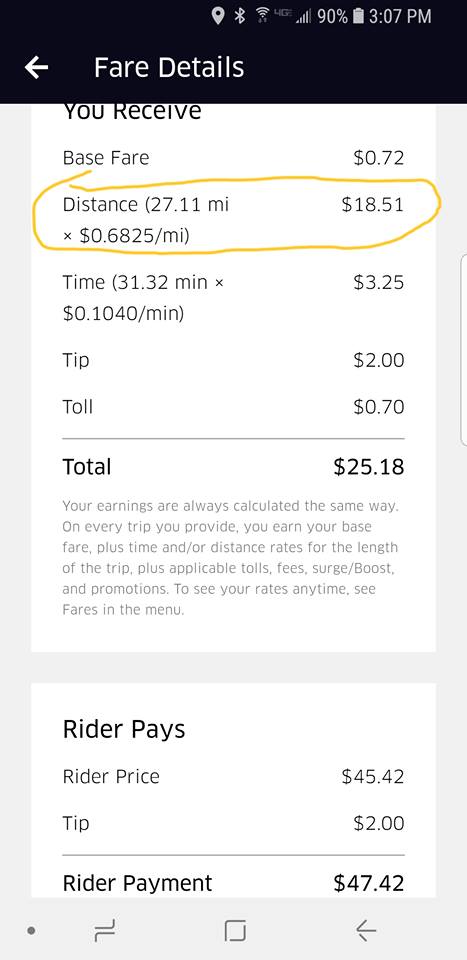This image appears to be a screenshot from a ride-sharing app displaying the fare details of a completed trip. The base fare is listed as $0.72. The trip covered a distance of 27.11 miles, calculated at a rate of $0.68 per mile, totaling $18.51. The trip duration was approximately 31.32 minutes, incurring a time cost of $3.25. Additionally, the fare includes a $2 tip and a $0.70 toll, bringing the total fare amount to $25.18. 

Below these details, the rider's charges are shown: the rider price is $45.42, the $2 tip is reiterated, making the total rider payment $47.42. The difference between what the rider pays and what the company charges the driver suggests that the driver earns approximately $20.18 from this trip. This detailed fare breakdown helps the driver understand their earnings and the amounts deducted for the company's charges and additional fees.